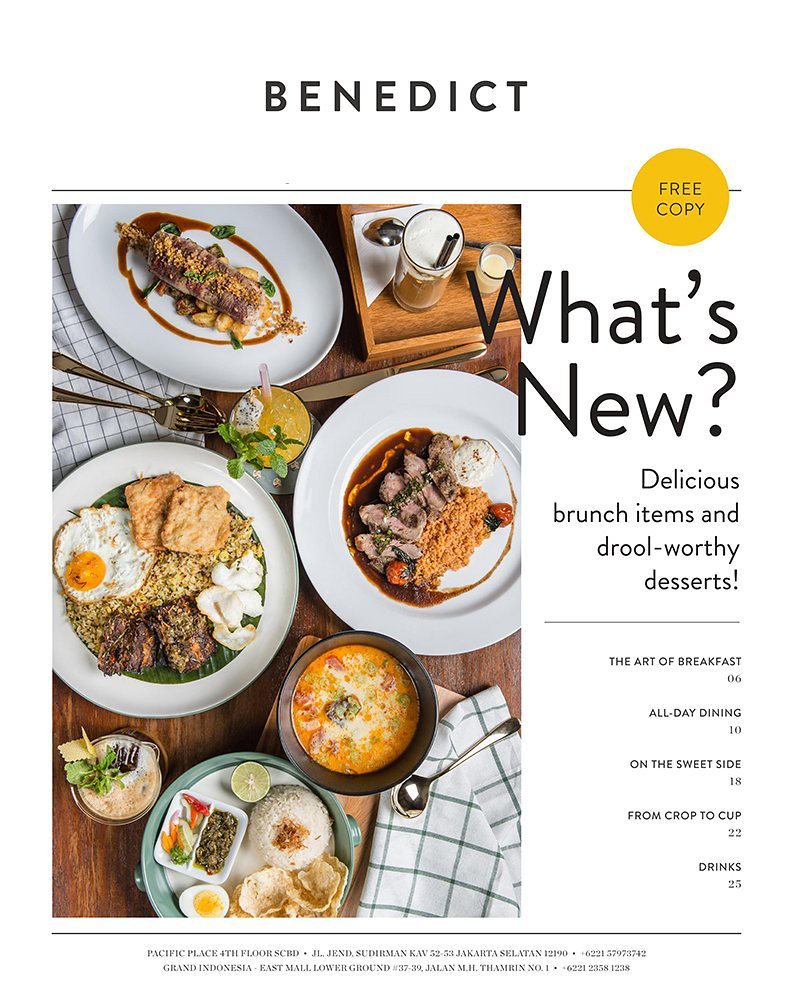The image is a detailed page that appears to be from a menu or a promotional flyer. It prominently features the word "Benedict" at the top, set in black text against a white background. To the right, a yellow circle contains the words "free copy" in black. Below this, the text "What's new? Delicious brunch items and drool-worthy desserts" stands out, followed by a list which includes "The art of breakfast, 6. All day dining, 10. On the sweet side, 18. From crop to cup, 22. Drinks, 25."

Accompanying the text, there is a beautifully photographed spread of various food items, captured from a top-down perspective. The table is adorned with a range of dishes: one plate features eggs, hash browns, and meat; another has sushi with a mound of rice; a bowl of soup is visible, and there's a plate with a meat dish covered in gravy. Additionally, a latte with two straws, two smaller bowls possibly containing soups or dips, and scattered spoons are part of the arrangement. The table is set with silverware and checkered napkins, adding a touch of style. The color palette of the image includes black, white, silver, green, gray, red, yellow, blue, orange, and brown, drawing attention to the vibrant and diverse dishes. The bottom of the page has small, somewhat illegible text, but parts of it appear to mention "Pacific Place fourth floor," "Jakarta," and "Grand Indonesia."